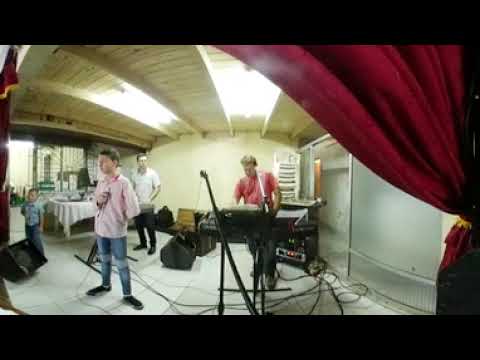The color photograph depicts a three-piece band either practicing or performing in what appears to be a small restaurant with a cozy atmosphere. Centrally framed, the band members stand in front of a red curtain that hangs prominently on the right side of the image. The leftmost band member, a young man around 20 years old, wears a short-sleeve pink button-up shirt, blue jeans, and black sneakers, holding a microphone and looking slightly to the left. Behind him is another band member dressed in a white t-shirt and black pants, standing with folded arms. To the right, a third musician stands in front of an electric keyboard, a guitar strap slung over his shoulder, wearing a red t-shirt and blue jeans, and looking down intently at his instrument. The scene includes cords and amplifiers scattered along the bottom of the stage area, a sliding glass door in the background on the right, overhead fluorescent lighting, and a light brown wooden ceiling. A young boy, about six or seven years old, can be seen to the far left of the image, adding a touch of casual intimacy to the setting.